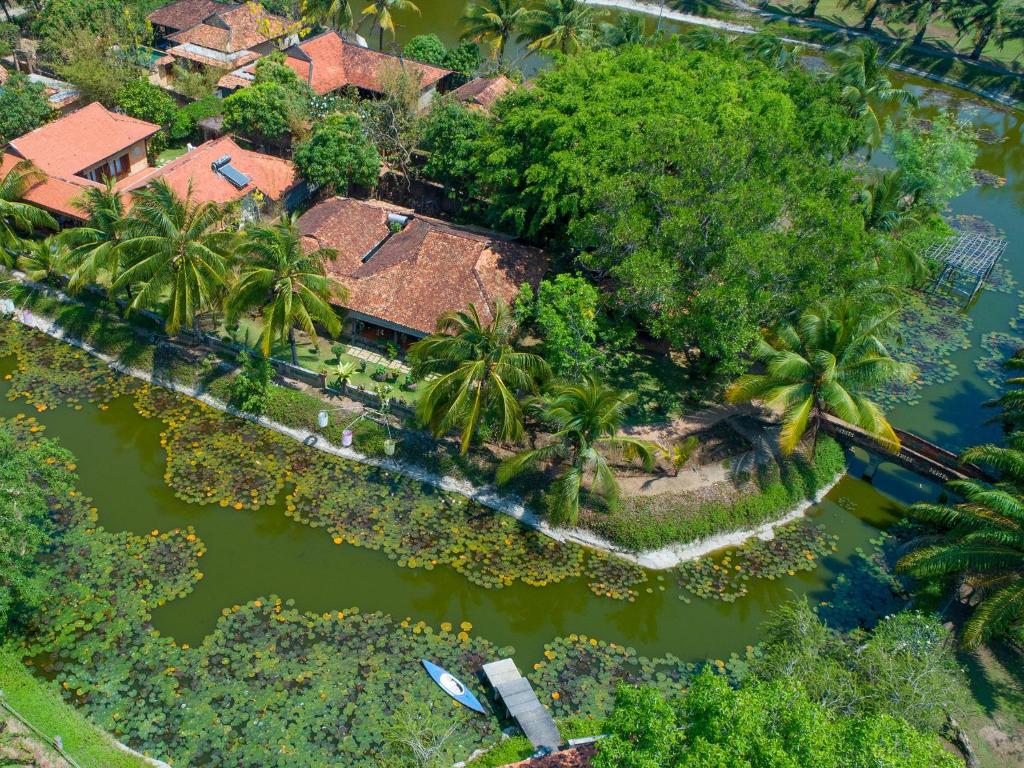This aerial photograph captures a small, densely packed island, most likely a village or resort, situated within a circular, swampy waterway that is reminiscent of the Florida Keys. The island is rectangular in shape and features six to seven houses with terracotta-colored roofs, partially obscured by a lush canopy of green foliage and numerous palm trees. Surrounding the island, the dark green, lily pad-covered water forms a narrow channel, making the area appear isolated yet connected to the mainland via a wooden bridge on the right side of the image. In the lower middle part of the photo, a green dock extends into the water, hosting a blue and white kayak. Dirt roads wind through the island, further adding to its rustic charm. The vivid reflections on the water indicate that the photo was taken during the daytime, enhancing the tropical atmosphere of this secluded, yet vibrant, oasis.